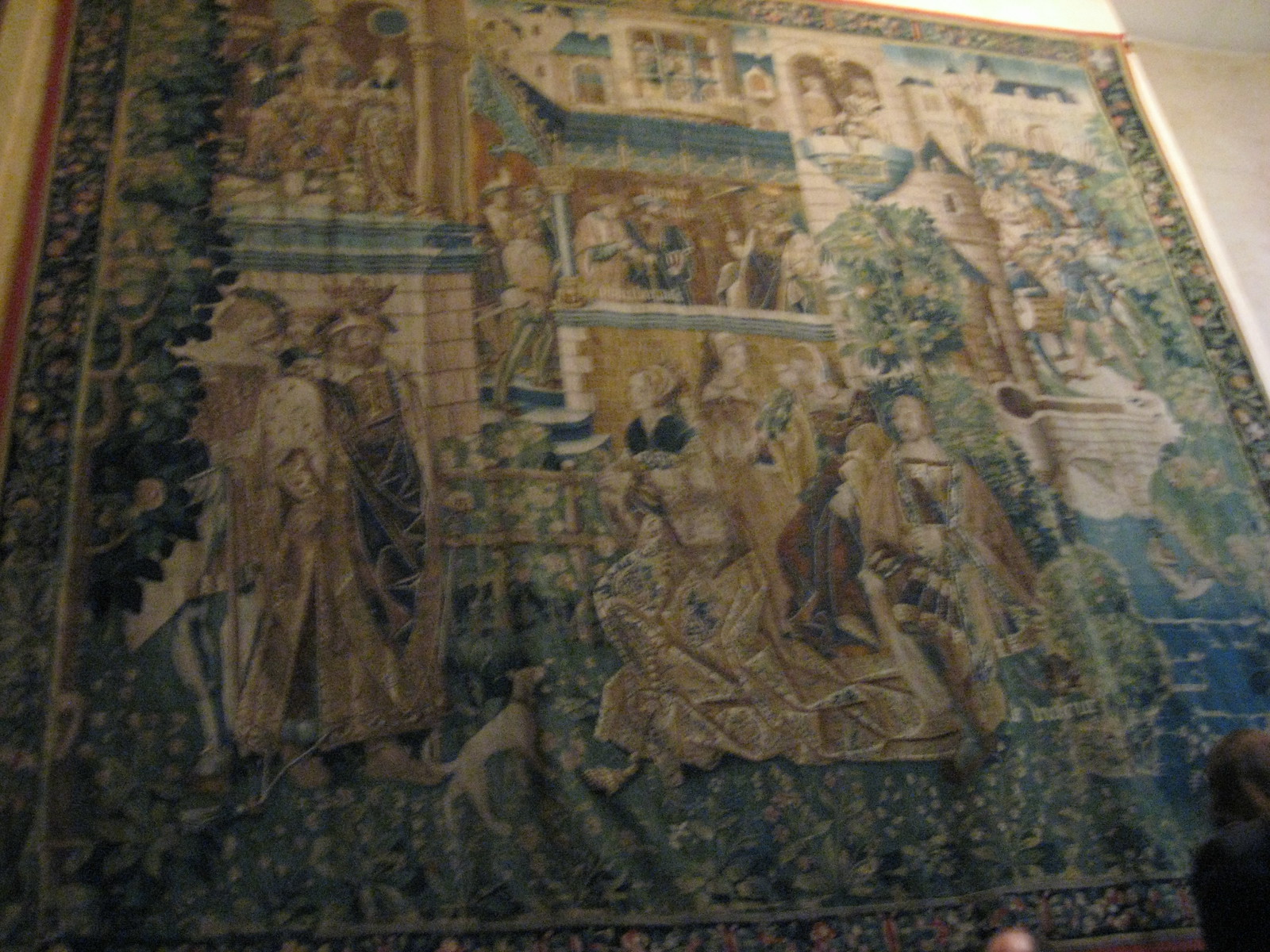The image depicts a large medieval-style tapestry, approximately 15 by 15 feet, nailed to a wall. The tapestry features a detailed scene with a blend of greens, yellows, and blues. It is framed by multiple borders—an initial gold border, followed by a red border, then a thick green border adorned with floral patterns, another gold border, and finally a red trim.

At the center of the tapestry, a grand two-story building, likely a castle, dominates the scene. The castle's walls are partially exposed, revealing various occupants: people can be seen inside the top floor on the left side, and on both the second and bottom floors in the middle section. 

In front of the castle, a king, distinguished by his crown, stands amidst a group of beseeching subjects. Nearby, two knights are positioned with a sense of vigilance, one on each side. To their right, a small dog with a brown head and white body is depicted looking up and to the right. Further to the right, three figures, one of whom is a woman in a long yellow dress, sit on a lawn.

The scene integrates elements of an outdoor garden, further enriched by the presence of shrubbery and a gray tower adorned with greenery attached to the castle's side. Despite some parts of the image being blurry, the vivid and meticulous portrayal of a medieval setting shines through, capturing a lordly figure surrounded by his people, various castle inhabitants, and the intricate landscape around them.